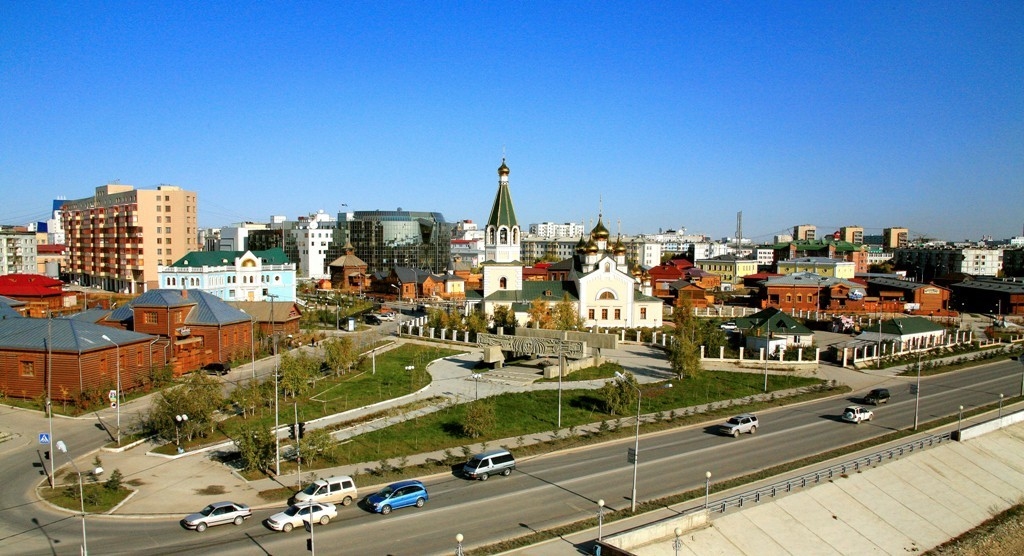The image depicts a photograph taken from a high vantage point, possibly from the top of a bridge or a tall building, overlooking a cityscape bathed in the bright blue sky. In the foreground, there is a diagonal road stretching from the right to the left, populated with various vehicles including a white car, black car, grey car, minivan, blue minivan, blue and white truck, silver car, and another white car, revealing a busy two-lane highway.

On the left side of the image, a notable teal-colored building, likely an apartment complex or condominium, stands tall alongside a brown building that could be a hotel. To the bottom left, where two roads intersect, forming a triangular point, there are patches of grass and several trees.

Across the middle section of the image, rows of brick and tan buildings with varying heights are visible, indicating a mix of residential and commercial structures. Standing prominently in the center background is a church with towering, pointy steeples that pierce the skyline.

The photograph is absent of any visible text or people, capturing a serene yet lively urban scene with its stone sidewalks and scattered greenery, further complemented by a distant hint of a helicopter hovering near the horizon. On the right side, a distinctive brick factory or industrial building adds to the architectural diversity of this quaint cityscape.